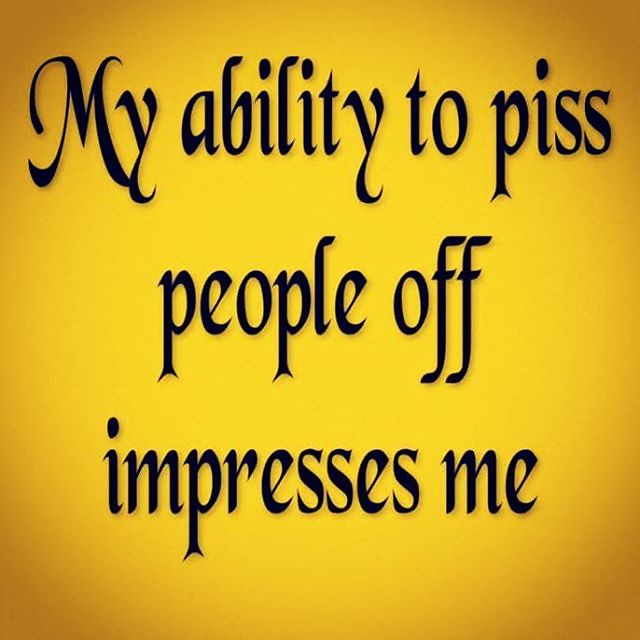The image features a simple, square sign with a gradient yellow background that transitions to darker mustard shades at the corners, creating a starburst effect. The centerpiece of the image is a large, black calligraphy-style text that nearly fills the entire frame. The text is split into three lines with ample spacing between them. The top line reads "my ability to peeve," the middle line says "people off," and the bottom line states "impresses me." The text is very prominent, almost touching the edges of the image, and there is no punctuation included.